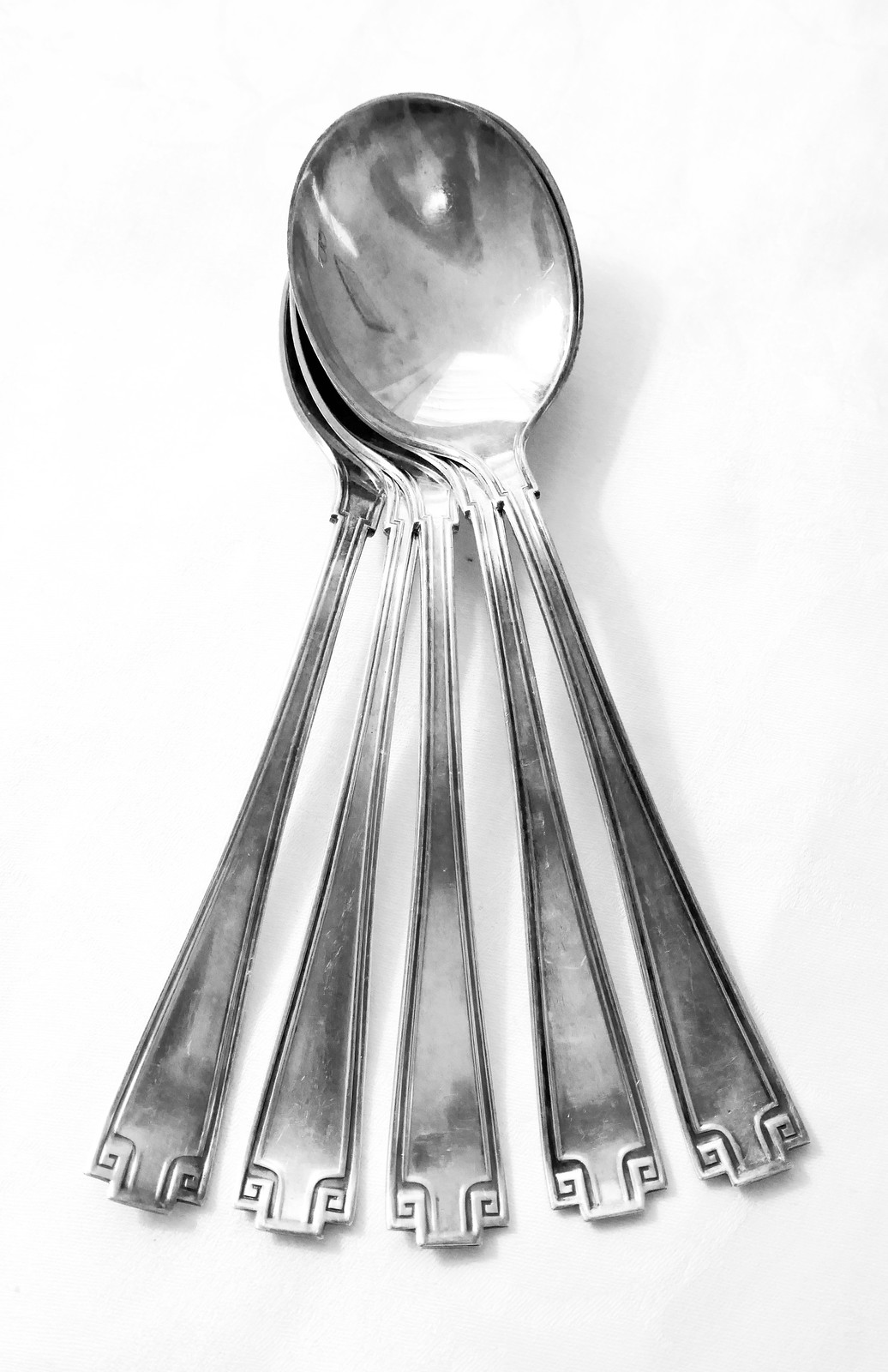This black and white illustration depicts a set of five shiny, reflective silver teaspoons arranged on a light white background. The bowls of the spoons overlap in the center, forming a piled configuration, while their narrow handles fan outwards to the sides, creating a visually balanced composition. The spoons cast a subtle shadow on the white surface, enhancing the depth and realism of the illustration. Each spoon features a distinctive handle design, characterized by a narrow base that widens towards the end, culminating in a blocky, ornate pattern with alternating rectangles and squares. The intricate shading and attention to detail suggest that the image might be created with pencils, and the fine gradations of light and shadow lend the scene a museum-like quality, possibly reflecting surrounding artwork.